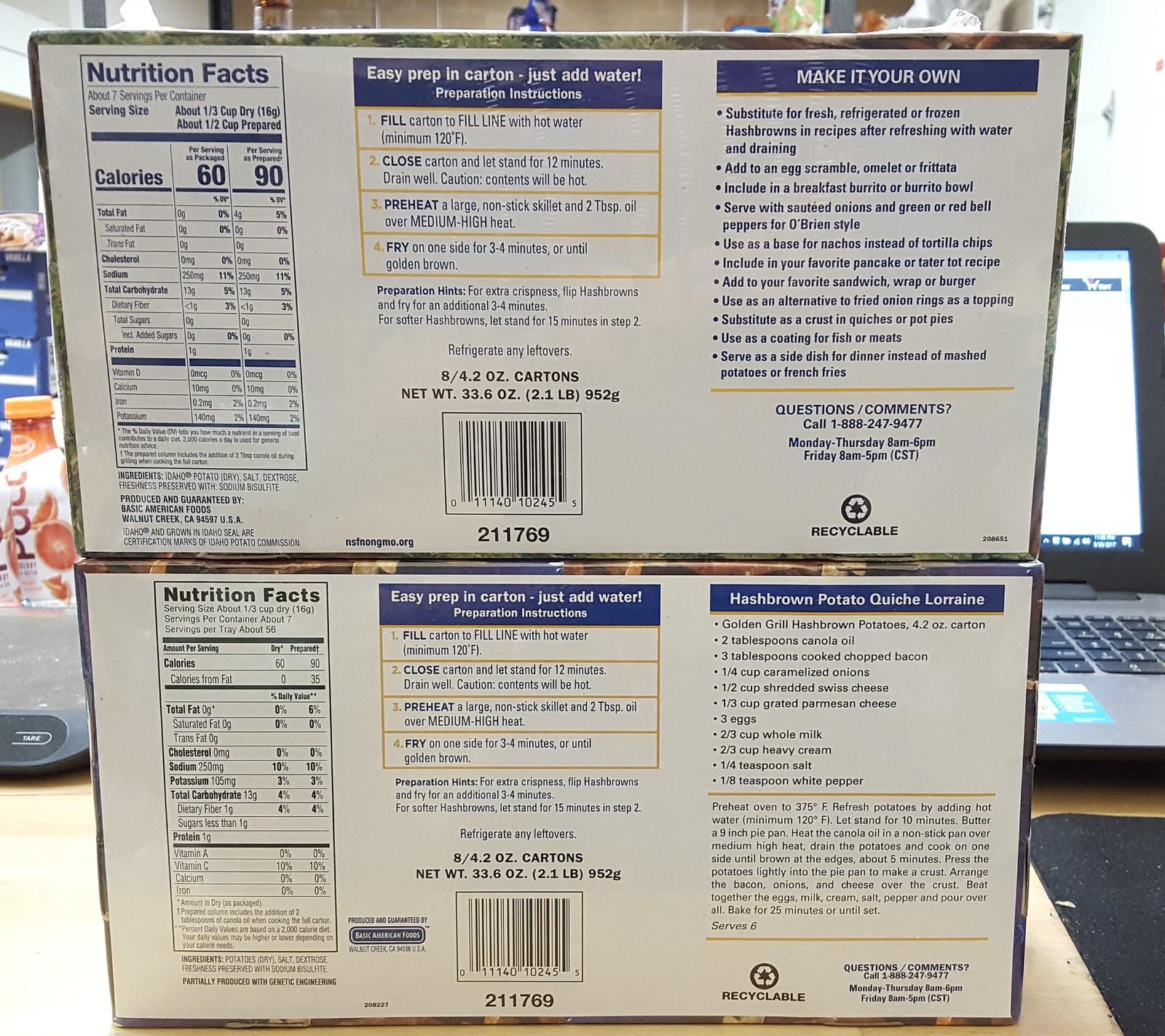This photograph captures the backside of two stacked packages, displaying their nutritional information. The focus is on the nutrition facts of the top package, prominently displayed on the left side. It indicates that the product contains approximately seven servings per container, with a serving size of about one-third cup dry or one-half cup prepared. In the center, the packaging provides easy preparation instructions, suggesting the addition of water directly into the carton. To the right, the package offers a suggestion to "make it your own" by substituting the product for fresh, refrigerated, or frozen hash browns in recipes. Near the bottom, it features the nsfnongmo.org certification and lists the ingredients: Idaho potato, dry, salt, dextrose, and sodium bisulfite for freshness preservation. The photo was taken indoors, evidenced by a laptop computer in the background and some drinks to the left side of the frame.